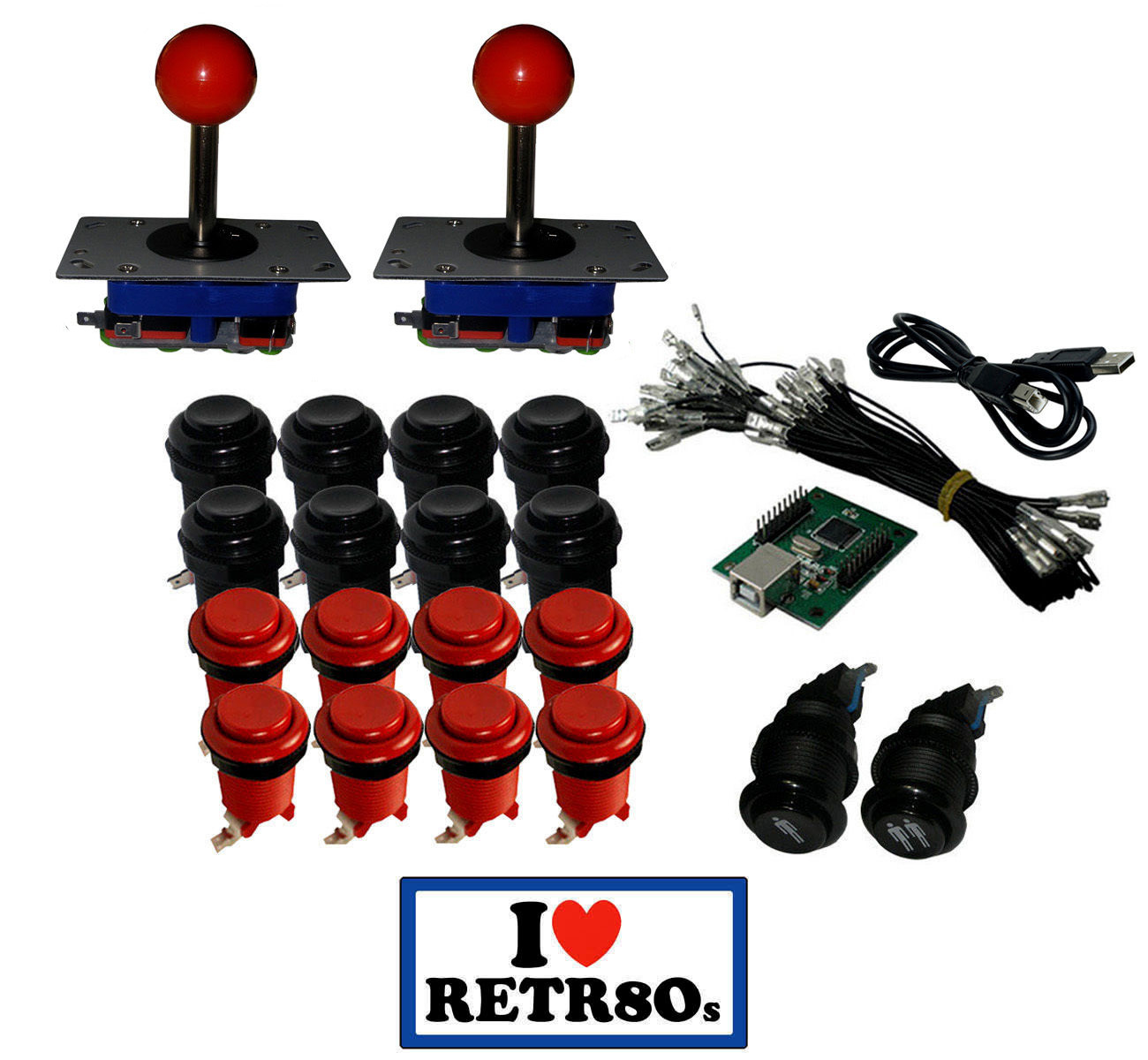This detailed photograph features a collection of retro 80s video game equipment displayed against a white background with a blue border. In the top left corner, two classic arcade joysticks are prominently positioned, each featuring a blue base with a black plate and a black joystick topped with a red ball. Directly below these joysticks, organized in two neat rows, are sixteen arcade-style buttons — the top row consisting of eight black buttons and the bottom row of eight red buttons, each with visible connectors underneath. 

To the right of the buttons, a green circuit board is visible, accompanied by various pieces of arcade equipment, including a bundle of cables and what appears to be additional connectors. A small chip, likely a motherboard-style component for programming, is also present. Additional items include what seem to be two black wireless earbuds and cables, possibly USB.

At the bottom of the image, a logo framed in blue contains the text "iHeartRetro80s," with the heart symbol in red, paying homage to the retro 80s gaming era. The arrangement and variety of components evoke a nostalgic sense of classic arcade and video game technology.